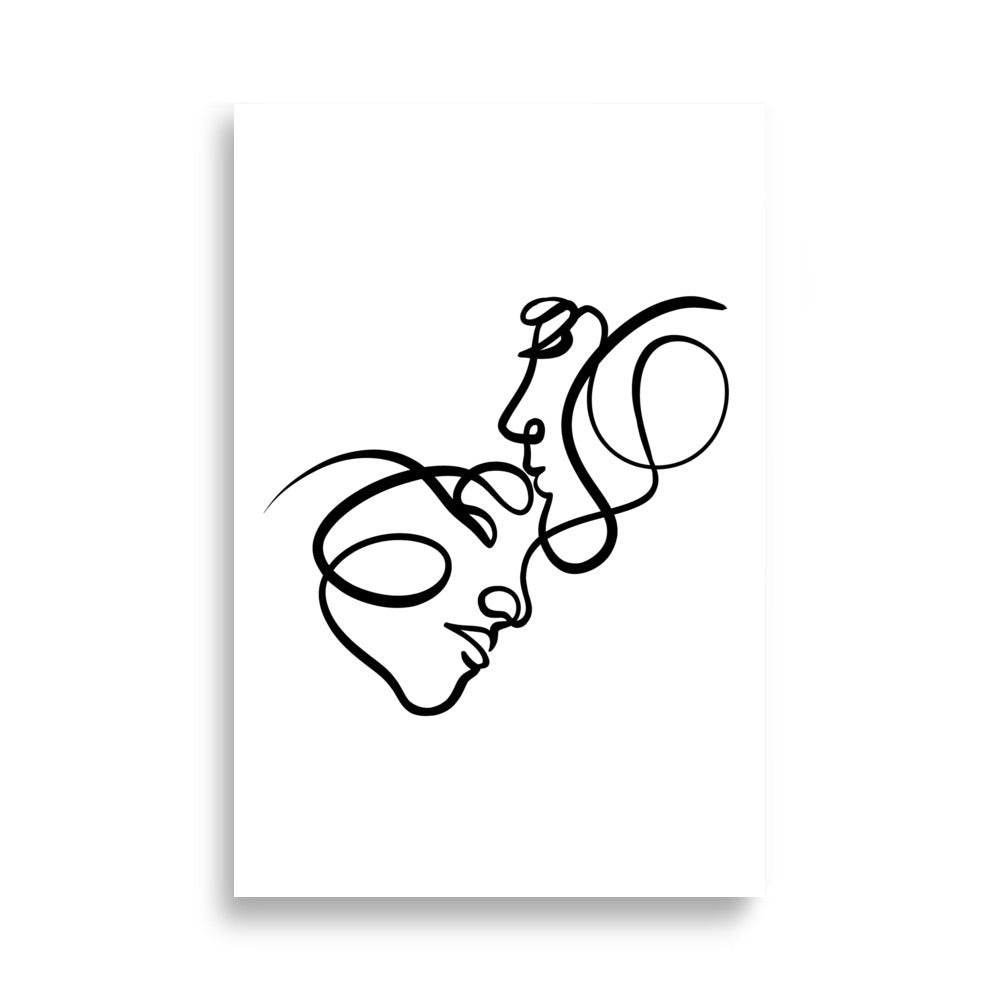The image is a white poster with a slight gray drop shadow on the left and bottom edges, enhancing the rectangular shape. It features a detailed and stylized pen and ink drawing, reminiscent of classic theater masks representing comedy and drama. The illustration is composed of intricate swirls and curves, seemingly created with a single continuous black line that forms the faces of a man and a woman. The man's face, identifiable by its male characteristics such as a prominent nose and lips, is in profile facing the left side, bending downwards as if to kiss the woman's forehead. The woman’s face, characterized by delicate features including closed eyes and softly outlined lips, nestles into the man's chest area and faces towards the right side of the image. Both figures have hair depicted by a series of elaborate swirls, enhancing the artistic and abstract nature of the drawing. The overall composition is simple yet deeply expressive, capturing a tender moment between the two figures through minimalist line art.